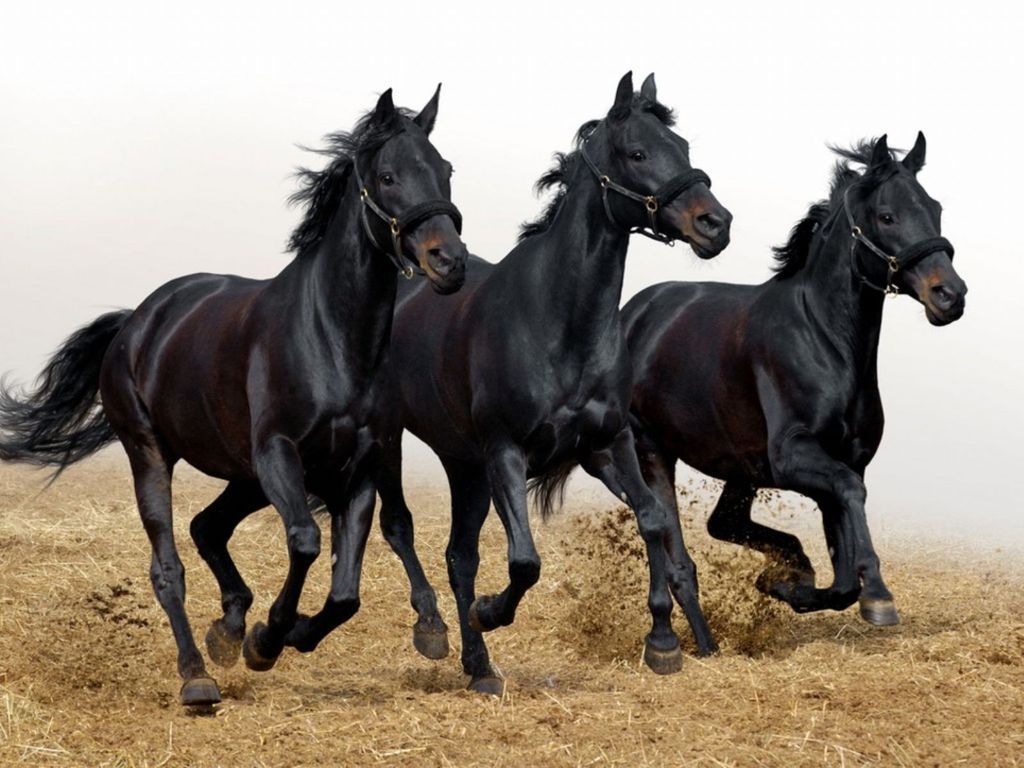The photograph depicts three black stallions, their glossy coats gleaming under a predominantly white sky that fades into light gray towards the horizon. These horses are captured mid-stride, trotting energetically in a direction akin to four o'clock. Positioned next to each other, you can see dirt and dead grass, resembling hay, being kicked up beneath their hooves, which are partly lifted off the ground. The horses' bridles are neatly fastened around their heads, and they all exhibit a subtle brown hue near their nostrils. Their flowing black manes and tails appear to be caught in motion, suggesting the wind's influence. Additionally, the tail of the horse to the far left is notably curved upward. The ground beneath them is a tan mixture of dirt and hay, further accentuating the dynamic movement of these spirited animals.